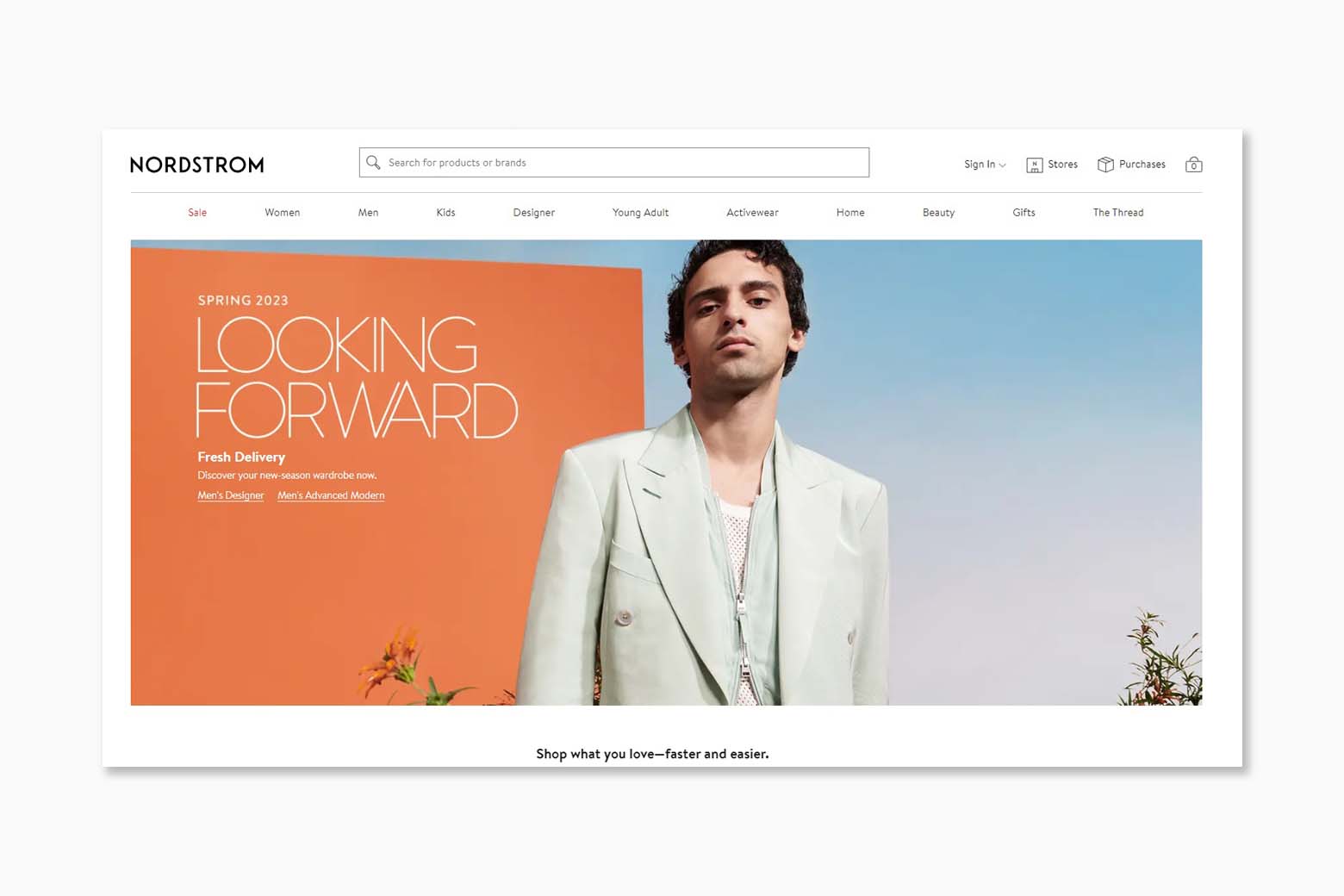Screenshot of Nordstrom's website featuring a promotional banner for their Spring 2023 collection. At the top left, the brand name "NORDSTROM" is displayed in all capital black letters. To its right, a search bar prompts users to "search for products or brands." Adjacent to the search bar, options for "Sign In," "Stores," and "Purchases" are available, accompanied by a shopping bag icon. Below this navigation bar, a horizontal menu lists various categories including Sale, Women, Men, Kids, Designer, Young Adult, Activewear, Home, Beauty, Gifts, and The Thread.

The main image showcases a tan man in his mid-20s to early 30s, with short wavy dark hair, full eyebrows, and sparse facial hair accentuated by a cleft chin. His expression is neutral, and he gazes directly at the camera. He is dressed in a mint green blazer over a white mesh fishnet shirt. An orange square behind him features text promoting the seasonal collection: "Spring 2023 Looking Forward Fresh Delivery Discover Your New Season Wardrobe Now Men's Designer Men's Advanced Modern Shop What You Love Faster and Easier." The scene is further adorned with flowers positioned to the left of the model, and a few additional flowers seen at the bottom right corner of the image.